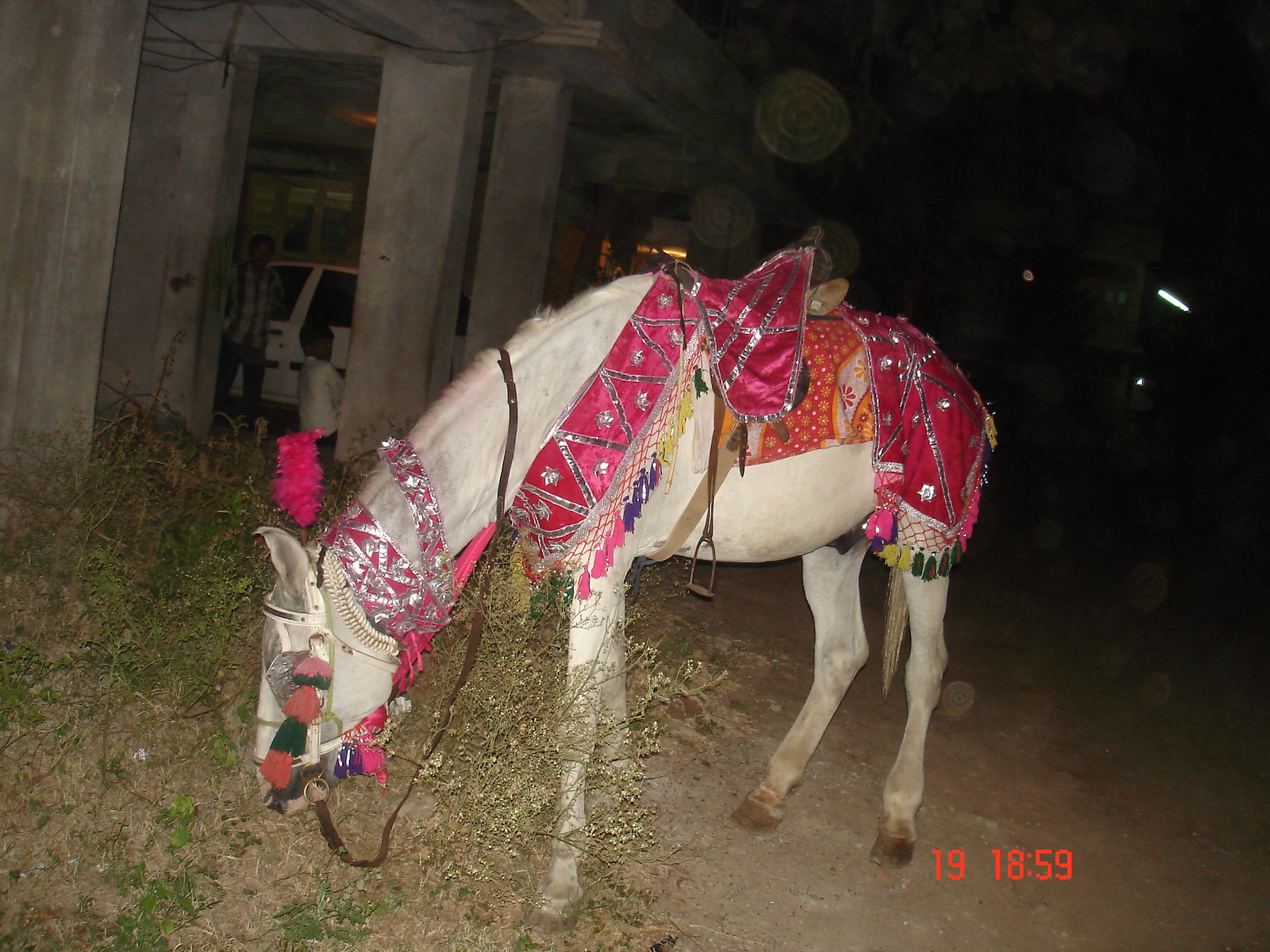The image depicts a white horse, potentially a donkey, taken outside at night, standing in a field with buildings in the background. The horse is centered in the photograph, oriented from right to left, with its head down as if grazing. It is adorned in intricate, multi-colored garments featuring pinks, reds, oranges, white, silver, and gold embroidery. The decorative attire includes an ornate saddle covered with a pink cloth, an orange cloth with designs beneath it, and a sash extending from its neck to its lower back. Additionally, a bridle with hanging decorations is visible on its face, including what appears to be a pink feather near the back of its head. Illuminated by the camera's flash, the foreground sharply contrasts with the dimly lit background, where a wooden building stands on the left and another building with faint lighting, housing two men, one standing and one sitting, is visible on the right. An orange timestamp reading "19 1859" is prominently positioned in the lower right corner of the image.